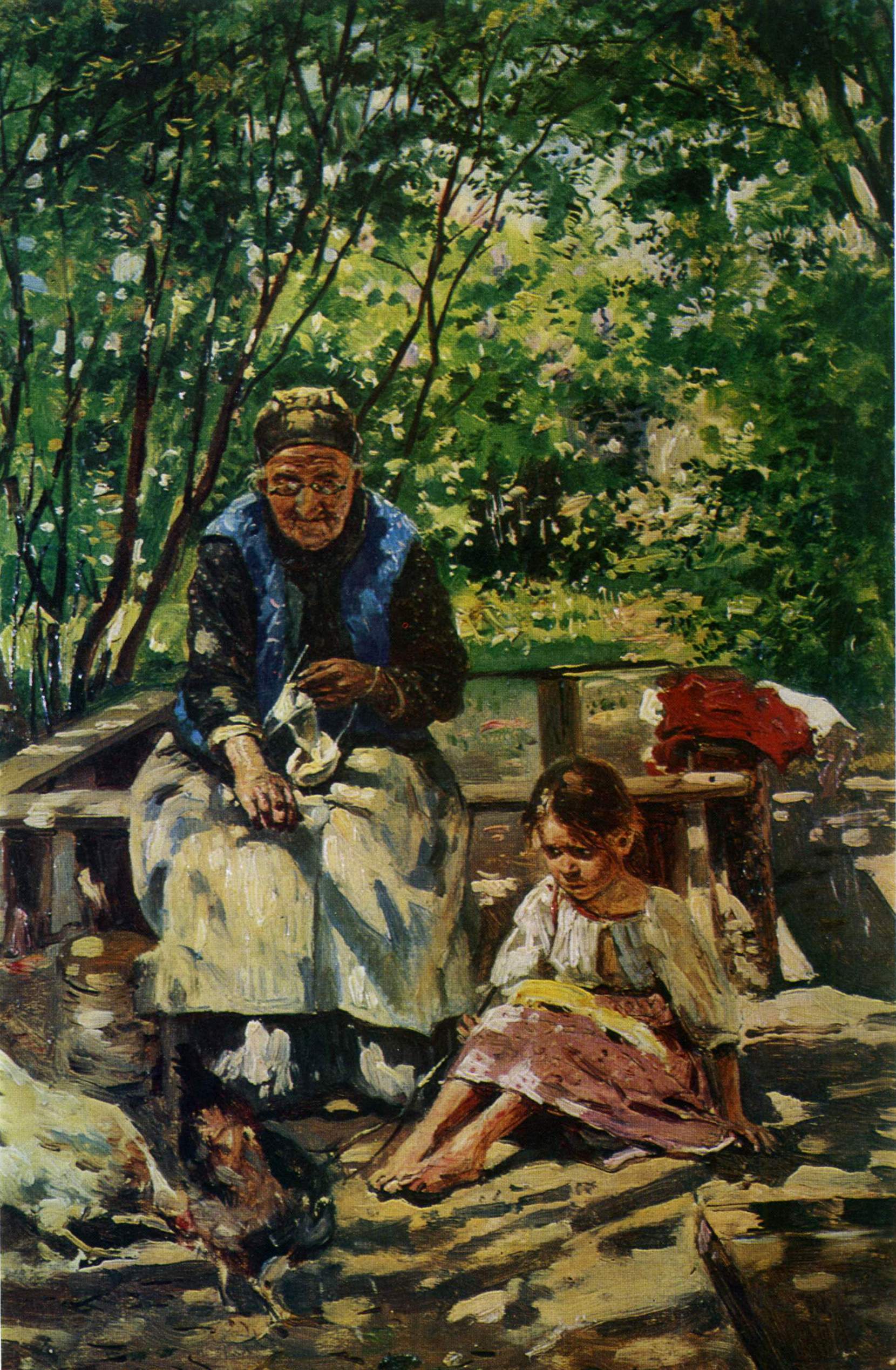The painting depicts an elderly woman and a young girl sitting outside in a sunlit, foliage-rich setting. The elderly woman, with her tan, wrinkled skin suggesting a life spent outdoors, wears a blue vest over a black, long-sleeved shirt speckled with white spots, complimented by a beige cover over her legs. She also dons a green cap, half-moon glasses, and appears to be knitting or sewing, her hands busily engaged. She sits on a chair amidst trees whose leaves range from bright green, illuminated by sunlight, to darker shades in the shadows.

At her feet sits a little girl clad in a pink skirt and a white top, her orange-brown hair pulled back in a ponytail, and her bare feet resting on the grass. The girl's wide eyes and fearful expression suggest she is reacting to the white and black chickens nearby. In addition to the lively foliage, painted in impressionistic strokes, there is a red and white object leaning on a bench in the backdrop. The scene exudes a tranquil, rustic charm, capturing a moment of daily life bathed in natural beauty.